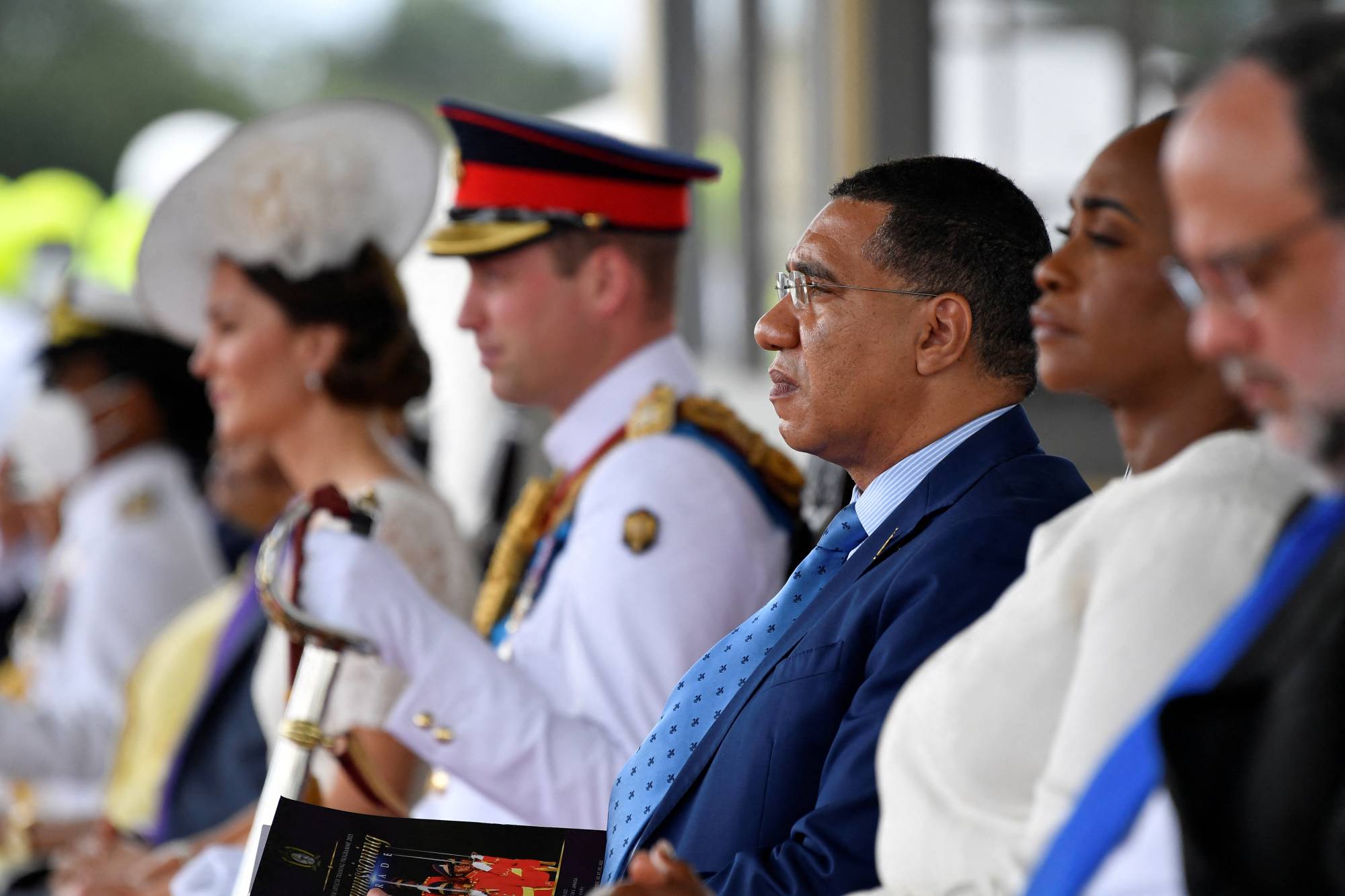In this detailed, outside photograph, a central figure, a man with brown skin, is dressed in a sharp blue suit paired with a blue tie adorned with black polka dots. He wears glasses, has short hair, and completes his look with a white collared undershirt. To his right stands a military personnel, donned in a white uniform and a distinctive black hat with a short gold brim and red rings, holding a sword while wearing white gloves. Positioned next to this uniformed man is a woman with short brown hair, adorned with a white hat decorated with flowers, and a white earring; she is dressed in a white dress indicating formal attire.

On the left of the central man is another woman, dressed in a simple white shirt, and on her left is a balding man with glasses and a goatee. He is attentively looking downward, dressed in a black suit and a blue tie. The far right of the image is somewhat blurry, revealing another person in a white shirt and a white and black hat, though details are indistinct. The background and secondary figures suggest the image depicts a formal or ceremonial event, possibly involving heads of state and military personnel from diverse ethnic backgrounds, set in broad daylight.